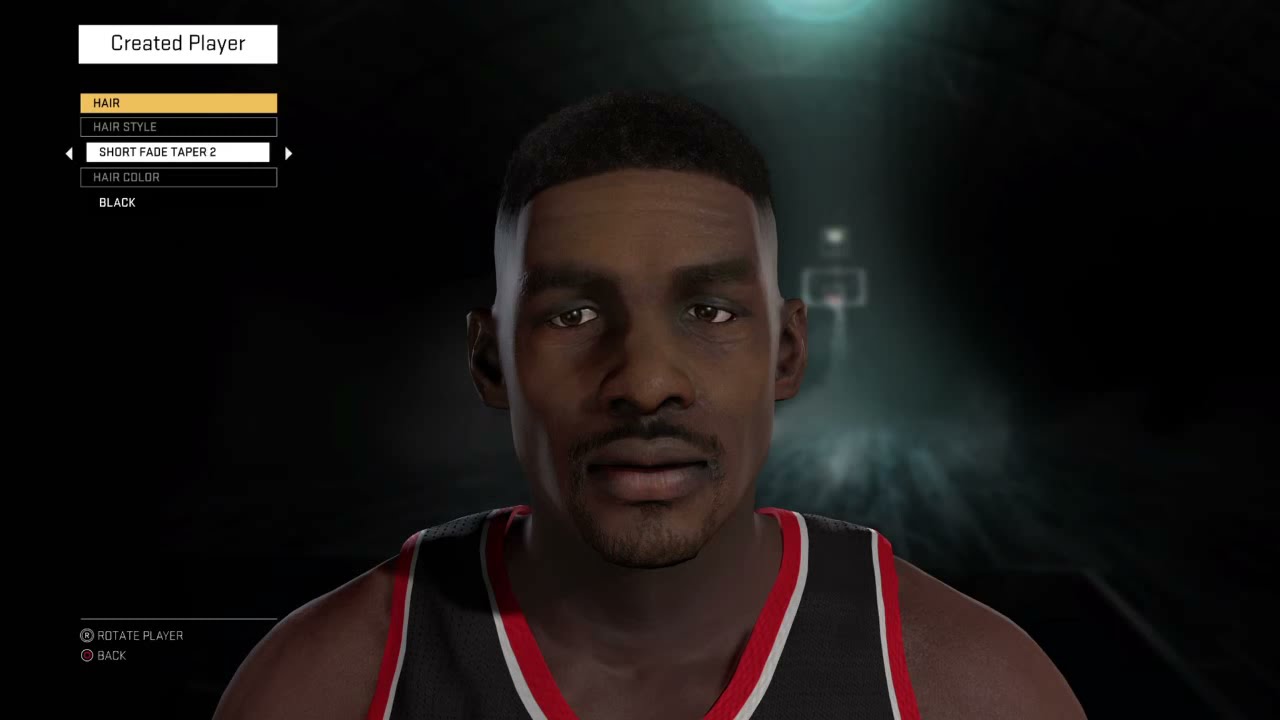In this image, a game character creation screen is displayed. The focus is on a player character being customized. In the top left corner, within a white field, the text "Created Player" is visible along with options for "Hair" and "Hairstyle," indicating the current choice as "Short Fade Taper" with the hair color set to black. At the bottom left, instructions for rotating the player using an arrow or right analog stick are shown, as well as a circle icon indicating the option to go back.

The character is depicted wearing sports attire in a striking color combination of black, red, and white. The background is predominantly dark, with a series of peach-colored lights providing illumination behind the player, adding a dramatic effect to the scene.